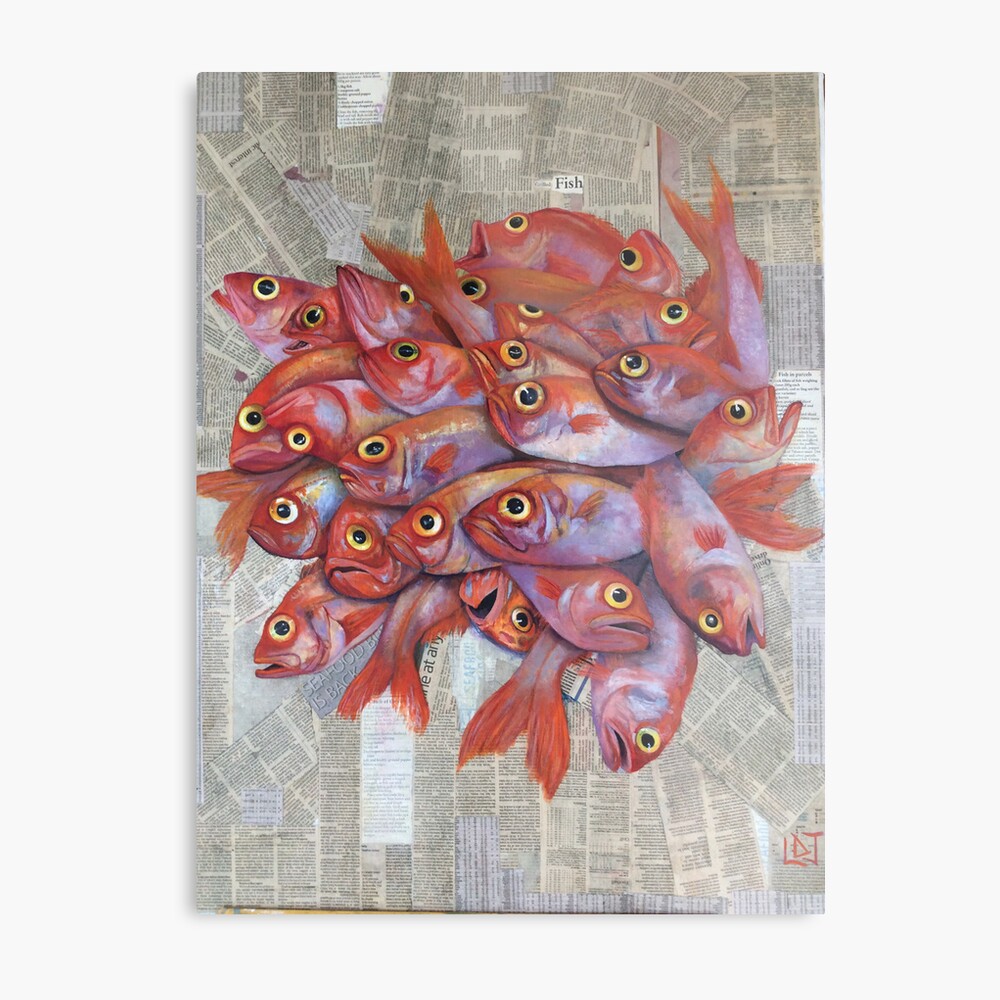This artwork is a vertically oriented, mixed media piece, prominently showcasing a centralized, tightly-packed circular formation of approximately 30 red fish. Each fish features a bright red head, lighter reddish-gray body, vivid red fins, and yellow eyes with black pupils, all facing in different directions – left, right, up, and down – evoking a sense of chaos or disarray. Expressions on their faces range from surprised to sad, and some have their mouths open, further amplifying a sense of distress.

The background starkly contrasts the vibrant fish with a monochrome patchwork of newspaper strips, cut into columns and rectangles, glued haphazardly in all directions. These papers vary in age and tone, from bright white to old and stained, creating a textured, chaotic backdrop. Among the newspaper clippings, the word "fish" is prominently cut out and glued at the top of the fish pile, adding a literal element to the visual narrative.

At the bottom right corner of the canvas, the initials “LDJ” appear in bold red, possibly indicating the artist's signature. This combination of elements – the vivid red fish against the fragmented, black-and-white newspaper background – creates a striking and thought-provoking piece.